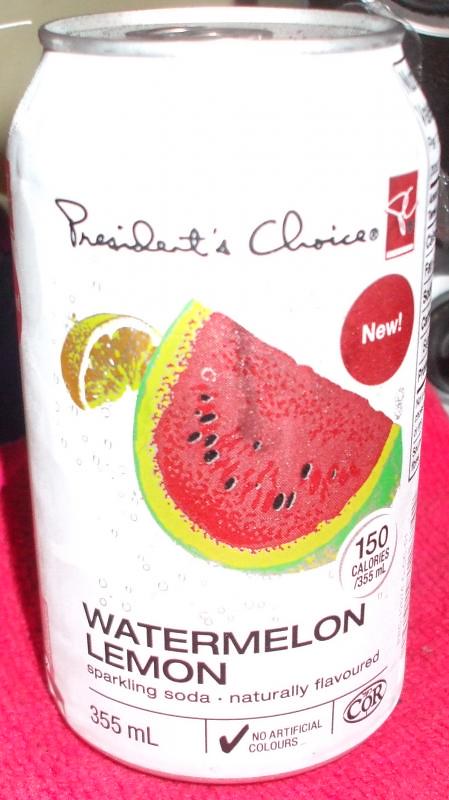In the image, there's an aluminum can prominently placed on a vivid, bright pink cloth. The background is a dark concrete wall, which provides a stark contrast to the colorful elements in the scene. The can itself is white and features distinctive branding elements. At the top of the can, "President's Choice" is printed in black letters. Just below this, there is a large, round red circle with the word "NEW" in bold white letters, indicating the product's novelty.

The can's design includes eye-catching illustrations of a yellow lemon slice and a red watermelon slice with black seeds and a green-yellow rind. The illustrations visually convey the flavors of the drink. Below these images, in bold black letters, the product is described as "Watermelon Lemon Sparkling Soda" and is noted to be "Naturally Flavored." Toward the bottom of the can, it states that the beverage contains 150 calories. The composition of the scene, with the bright pink cloth and dark background, effectively draws attention to the can, making its details stand out vividly.